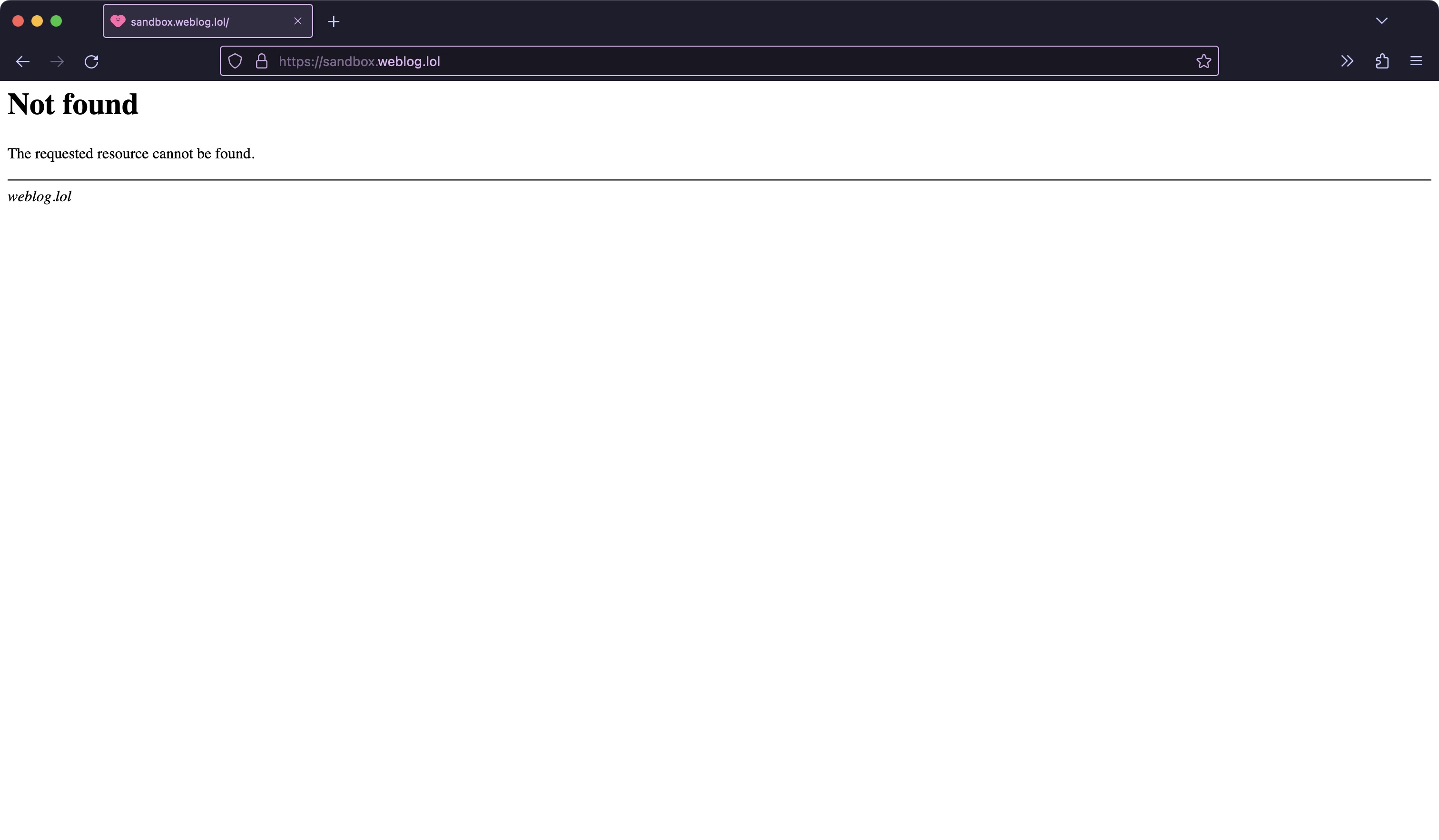The image predominantly features a blank white screen with no visible borders or edges. Along the top of the screen is a prominent message reading “Not Found - The requested resource cannot be found.” Beneath this message is a horizontal line spanning from left to right, indicating the URL “weblog.something.”

At the very top of the image, a black address bar is visible. In the far left corner of this bar, there are three side-by-side circular buttons—red, yellow, and green. Directly below these circles are three navigation icons: a back arrow, a forward arrow, and a refresh button.

At the top of the browser window, there is an open tab displaying an icon of a pink heart on its left side, labeled "sandbox.something." To the right of this tab is a plus sign for opening a new tab. Below these elements is a long address/search bar containing the text “http something weblog.”